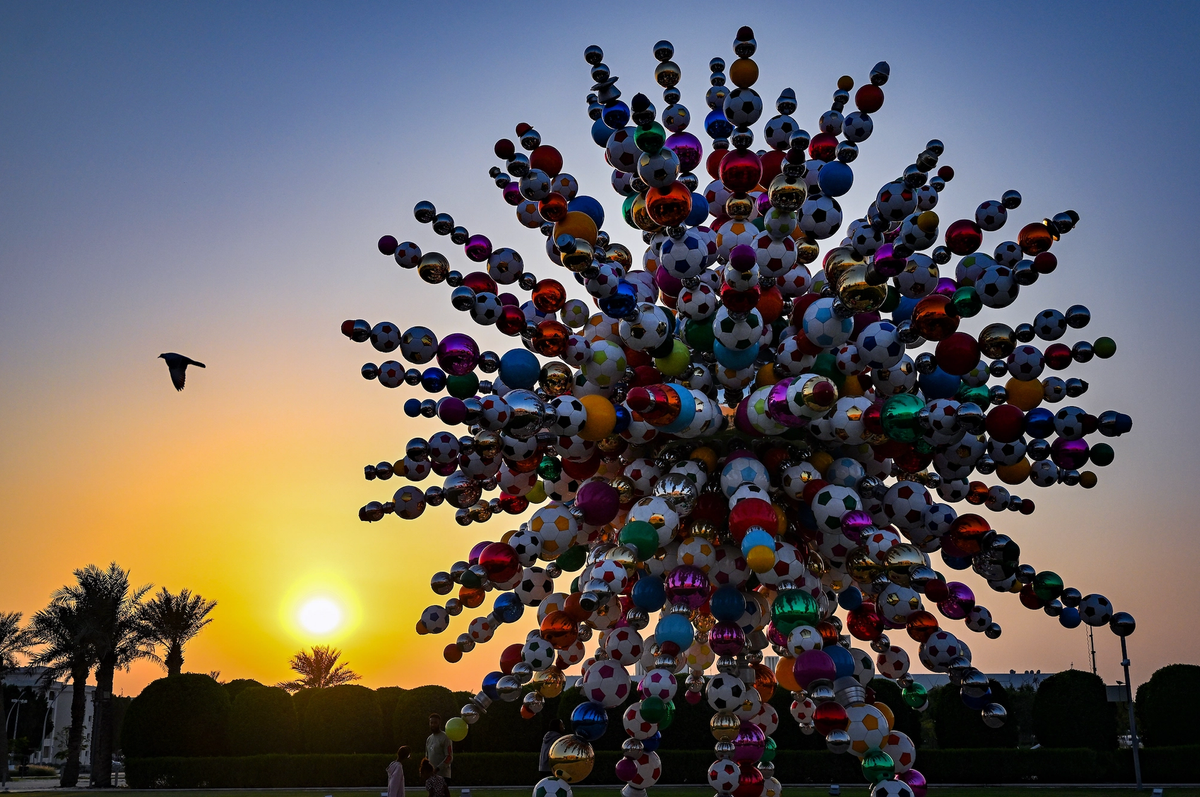The image depicts an intricate outdoor sculpture composed of various colored objects resembling soccer balls or plastic balloons. These multicolored balls—shiny blue, red, traditional black and white soccer balls, and orange and white variants—are mounted on what appear to be spikes or stick-like structures, creating an effect reminiscent of a spherical tree with branches extending outward. The sculpture stands prominently in a park-like setting, with the backdrop of a stunning sunset illuminating the sky with hues of orange, yellow, and a darkening blue. The setting sun casts shadows on the surrounding palm trees to the lower left, a bird mid-flight on the left side of the image, and obscured vehicles in the background. The entire scene is imbued with a striking interplay between the colorful sculpture and the serene, shadowed surroundings.